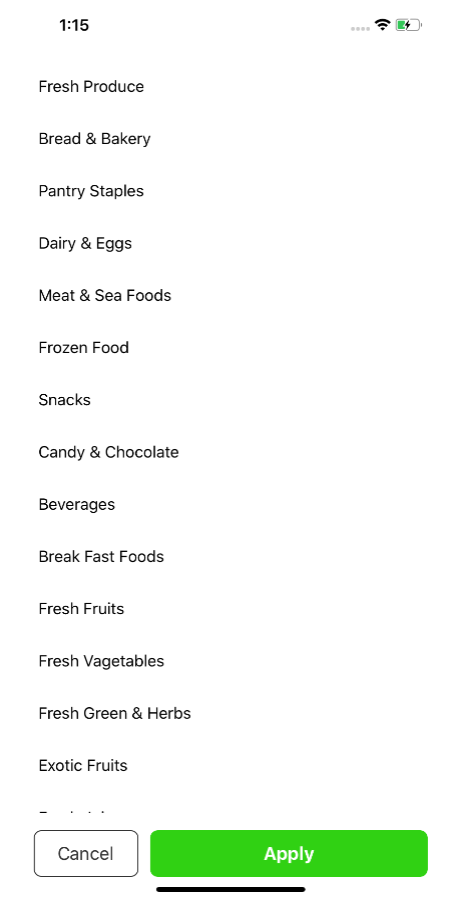This image features a white background with black text and various icons. At the very top, in black text, the time is displayed as 1:15. To the right of the time, there is a Wi-Fi signal icon and a battery icon that appears half full, indicated by a green fill in the lower half.

Beneath these icons, the image lists several categories of products, each in black text on the white background. The categories are:

1. Fresh produce
2. Bread and bakery
3. Pantry staples
4. Dairy and eggs
5. Meat and seafood
6. Frozen food
7. Snacks
8. Candy and chocolate
9. Beverages
10. Breakfast foods
11. Fresh fruits
12. Fresh vegetables
13. Fresh greens and herbs
14. Exotic fruits

At the very bottom left of the image, there is a rectangular box outlined in thin gray, containing the word "Cancel" written in gray text. To the right of this box, there is another rectangular box, this one filled with green and having the word "Apply" written in white text. Below these boxes, there is a thin black line. Additionally, beneath the last word on the list, there are small dots and a line suggesting the presence of more text beyond what is visible.